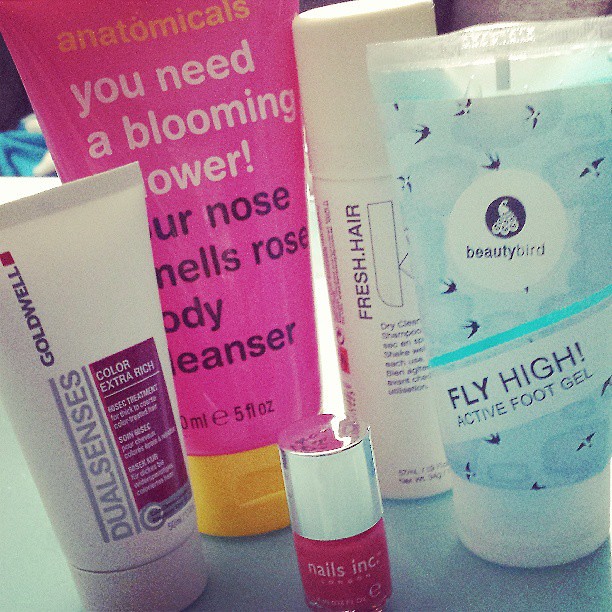This photograph, taken indoors, captures a close-up of various body and skincare products neatly arranged on a countertop, with prominent emphasis on their colorful packaging and labels. Starting from the left, there's a smaller white squeeze bottle labeled "Dualsenses Goldwell" with magenta accents, featuring "Color Extra Rich" in gray text and topped with a white cap. Slightly behind it, a large pink squeeze bottle stands out, marked "Anatomicals," with the text "You need a blooming shower. Your nose smells rose body cleaner" partially visible, capped with yellow. Next to it sits a slender white canister that likely has a roll-on or spray applicator, labeled "Fresh Air" in black text. Moving further right, there's a blue and white squeeze bottle from the brand "Beauty Bird," prominently displaying "Fly High Active Foot Gel" within a blue banner. At the forefront, there is a small bottle of pink nail polish labeled "Nails Inc," positioned in the center-left of the arrangement. The aesthetic interplay of colors and text on the bottles creates a visually engaging composition that highlights the diversity of everyday personal care items.